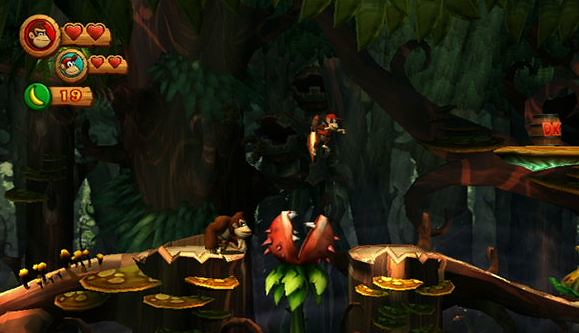This image is a still from the video game Donkey Kong, featuring a dark, forest-like background with shades of black and green. The scene includes various elements typical of the game. In the upper left corner, there's a detail of the game interface showcasing two monkeys. The larger monkey's face appears alongside two red hearts, indicating lives or health status, while the smaller monkey, wearing a red cap, is also displayed with two hearts.

Amidst the lush green trees, which have their trunks colored in black to emphasize the dark setting, there's a central figure—a bright, red, and gold animated character. This character is likely interacting with a complex scene around them. To the right, there's a red and green light fixture illuminating part of the environment.

On the ground, there's a tabletop scene where a red fish with green tentacles or tail and an open mouth is set, possibly suggesting some in-game interaction or objective. A small squirrel observes this setup, and it seems like pancakes are being served on the table. Additionally, trees and perhaps lily pads suggesting a water effect add to the immersive forest background.

Notably, a prominent feature is a red, spiky plant situated centrally, which resembles a carnivorous plant with teeth, ready to eat anything that falls into it. The smaller monkey is depicted attempting to jump over this perilous plant using a jet pack with fire emanating from it. Above these, various UI elements include a gold bar with the number 19 and green circle containing a yellow banana, further enhancing the typical game details and objectives.

This detailed and dynamic composition perfectly captures the adventurous and whimsical essence of the Donkey Kong game.